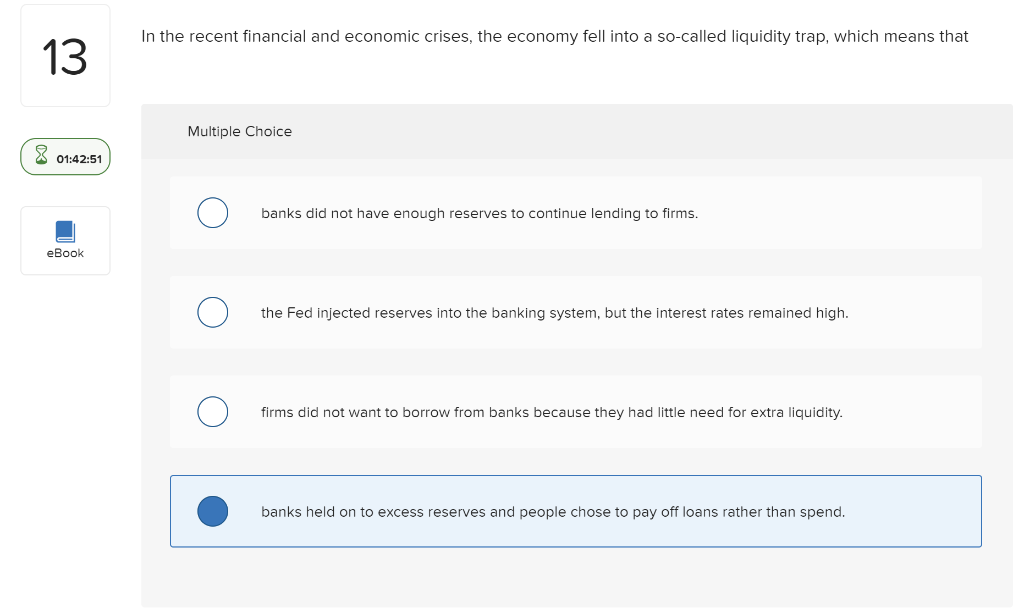The image is a widescreen, borderless screenshot of a financial and economic test. At the top left corner, there's a small, portrait-oriented, gray box with the number "13" displayed in black. Adjacent to this box, a sentence reads: "In the recent financial and economic crises, the economy fell into the so-called liquidity trap, which means that..."

Directly below the sentence, there is a horizontal gray box containing four radio buttons, each accompanied by text options. These radio buttons reside within a lighter gray box and are white inside. The text options presented are:

1. "Banks did not have enough reserves to continue lending to firms."
2. "The Fed injected reserves into the banking system and interest rates remained high."
3. "Firms did not want to borrow from banks because they had little need for extra liquidity."
4. "Banks held on to excess reserves and people chose to pay off loans rather than spend."

The fourth option is highlighted in blue, indicating it has been selected, with the radio button filled in a matching blue color.

Just below the number "13" in the upper section, there's an oval-shaped button featuring an hourglass icon with green sand at the bottom. The displayed time next to this icon is "1:42:51." Further below and to the left, there's a gray box with an icon of a blue book labeled "e-book."